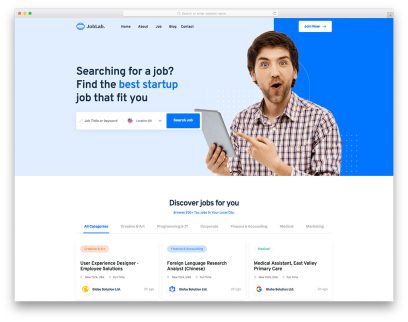A screenshot of a job search website's home page. The top section, which features a gradient background transitioning from darker blue on the right to lighter blue on the left, prominently displays the tagline, "Find the best startup job that fits you." Below this tagline, there are two search fields provided for users to input their job preferences. 

A central part of the image shows a stock photo of a man in a plaid shirt, holding a tablet and looking directly at the camera with a surprised and excited expression. 

As you scroll down the page, there's a section titled "Discover jobs for you," presenting various job listings including positions like User Experience Developer, Foreign Language Research Analyst specializing in Chinese, and Medical Assistant. 

The bottom half of the page has a clean, white background, contrasting with the blue gradient above, lending a clear and organized appearance to this generic job site which might cater to a wide range of professional opportunities, possibly both online and offline roles.